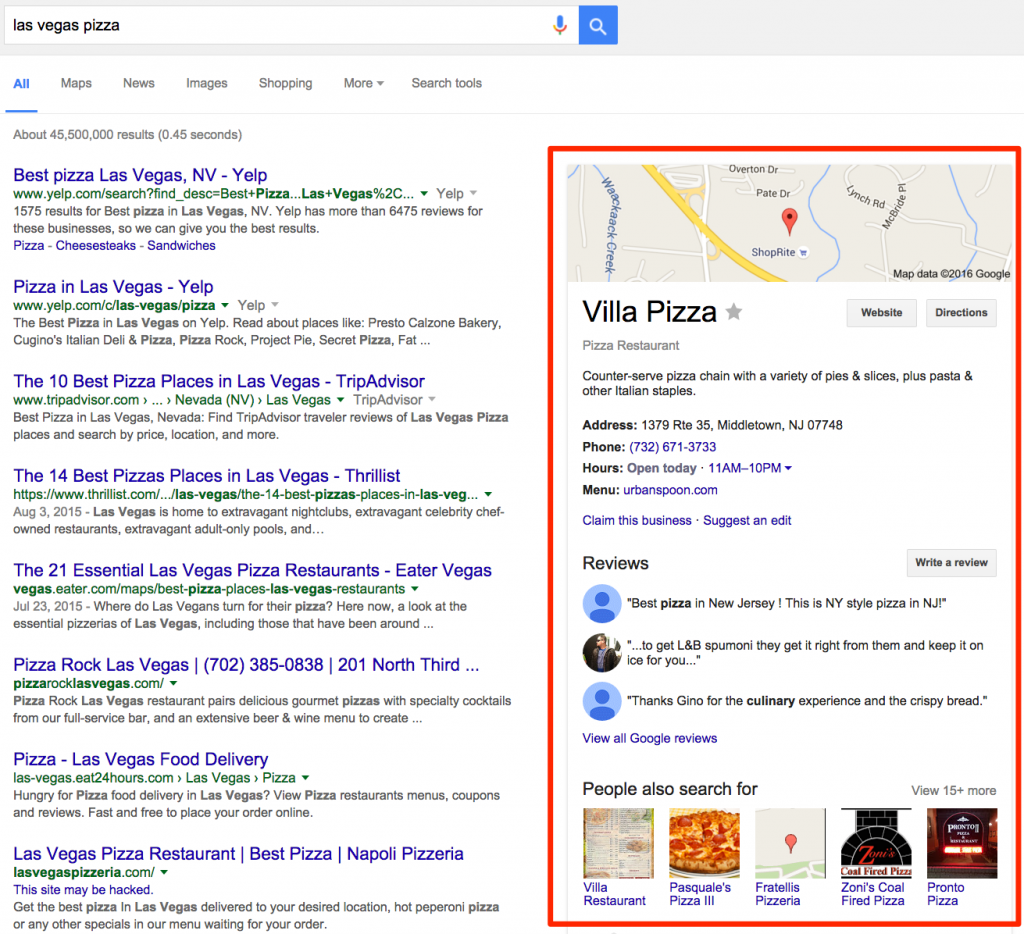Screenshot of Google Search Result for Villa Pizza

The screenshot features a highlighted search result, outlined in a red rectangle, for "Villa Pizza" located in Middletown, New Jersey. This listing includes a small map snippet with a red pin indicating the restaurant's location near ShopRite, Pate Drive, Lynch Road, and McBride Plaza. The map data is attributed to Google, 2016.

Key details about Villa Pizza are prominently displayed:
- **Name:** Villa Pizza
- **Type:** Pizza restaurant
- **Description:** Counter-serve pizza chain offering a variety of pies and slices, plus pasta and other Italian staples.
- **Address:** 1379 Route 35, Middletown, New Jersey, 07748
- **Phone Number:** (732) 671-3733
- **Hours:** Open today from 11 a.m. to 10 p.m.
- **Menu:** Available on urbanspoon.com
- **Features:** Options to claim the business or suggest edits

The image includes reviews from patrons, one of which states, "The best pizza in New Jersey. This is NY style pizza in NJ." Another review mentions, "To get L&B Spumoni, they get it right from them, and keep it on ice for you." A third review thanks "Gina for the culinary experience and the crispy bread." There is also a link to view all Google reviews, albeit slightly obscured by a purple highlight.

Below the detailed Villa Pizza information, there are suggestions under "People also search for" which include:
- Villa Restaurant
- Pasquale's Pizza 3
- Fratelli's Pizzeria
- Zoni's Coal Fired Pizza
- Pronto Pizza

The comprehensive details provided make it easy for potential customers to gather essential information about Villa Pizza and nearby alternatives.